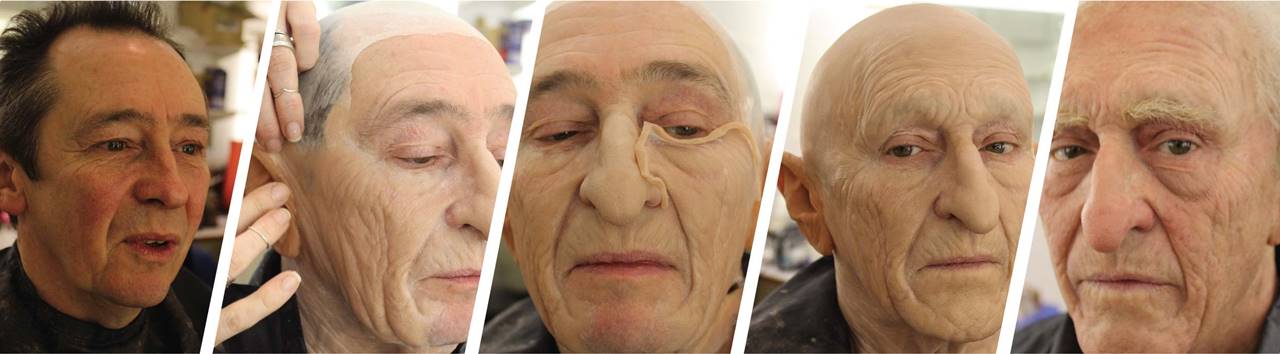The image is a series of five color photos depicting the transformation of a younger man into an elderly character through the application of a detailed prosthetic mask. The sequence begins with an actor in his 50s with dark hair, looking to the right. In the subsequent image, a person's hands, possibly belonging to a woman with a wedding ring, are seen working around his ear, applying parts of the old man mask. Each progressive shot reveals more of the transformation: the third image is a close-up of the mask being applied below his eyes, showing deep wrinkles and significant aging effects. By the fourth image, the actor appears bald with a fully applied mask, revealing a very wrinkled face and sparse gray hair. In the final photo, the actor is turned to the left, fully transformed into an elderly man with prominent wrinkles, grayish-white hair, and a look of concern, emphasizing the realism and detailed craftsmanship of the makeup process.